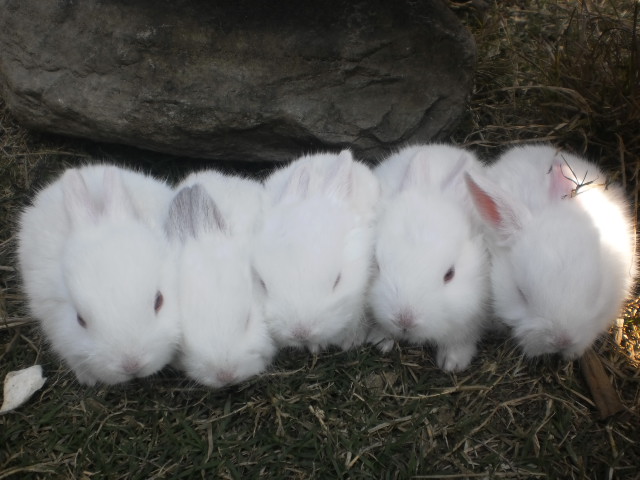This is a detailed photograph capturing five fluffy, white baby bunnies huddled closely together on grassy bedding. The rabbits are positioned under a rocky formation, which hangs down above them, creating a snug shelter-like ambiance. The surroundings are a bit dark, filled with shrubs and grassy debris. The endearing bunnies exhibit varying expressions: the first bunny on the left is wide-awake and gazes directly at the camera, the second is more snuggled in with its eyes closed, the third has its eyes partially open, the fourth looks alert with open eyes, and the fifth bunny, with its distinctively pink ears highly visible, is peacefully sleeping.